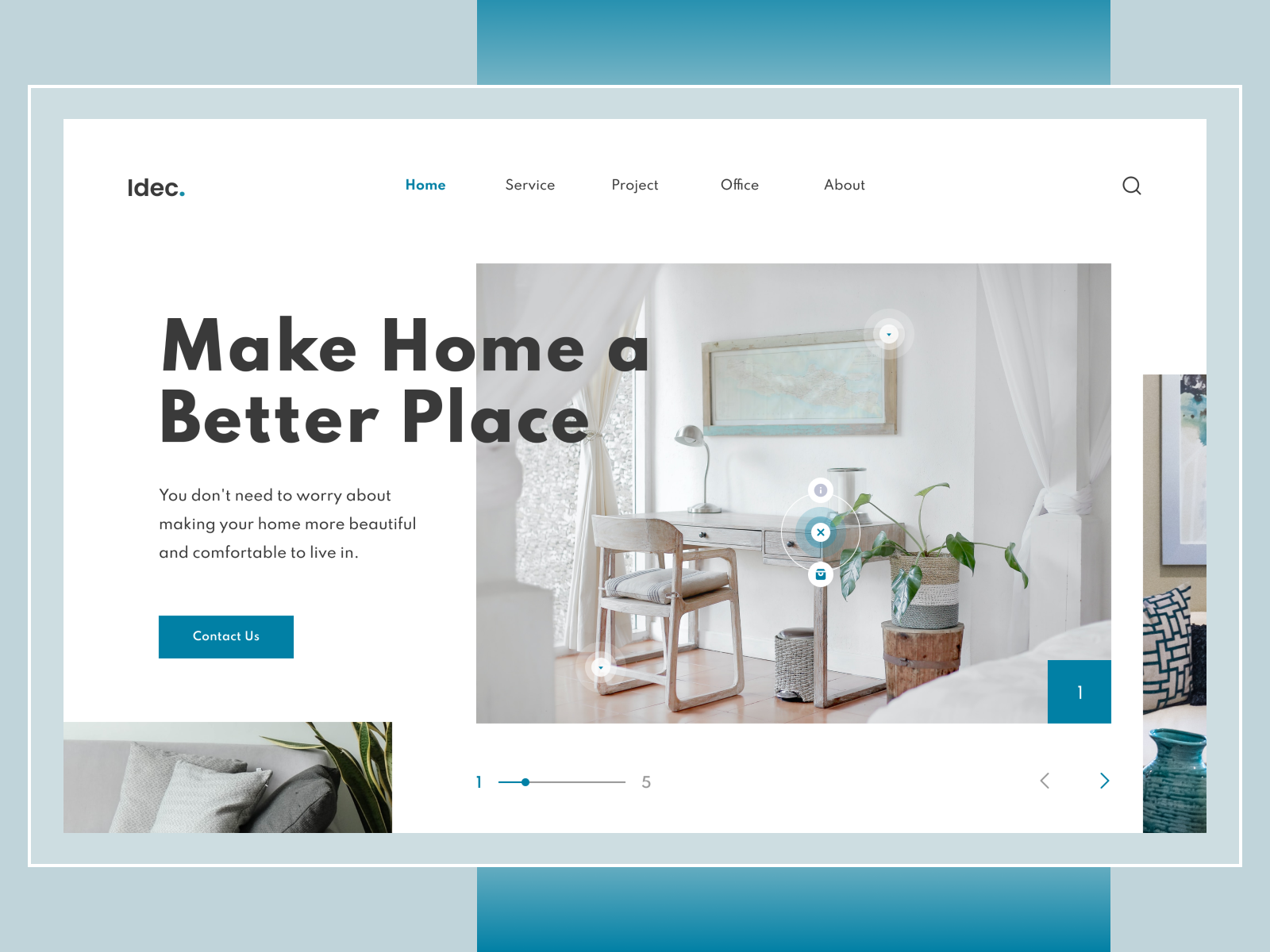This is a detailed caption for the described image: 

---

**A Visually Engaging Homepage Design**

The screenshot showcases the homepage of a website featuring a background composed of three blue stripes. The most prominent stripe, centered on the right side, exhibits a blue gradient that transitions from dark at the top and bottom to lighter in the middle. Adjacent to it on the left is a slightly narrower stripe in a pale blue hue, mirrored by an even thinner stripe on the right edge, sharing the same pale blue color. 

Superimposed on this is a thin white rectangular outline encapsulating a light blue pane. Nested within this frame lies the primary content area with a plain white background. Positioned in the top left corner, bold black text prominently displays the website name, "IDec," with the "I" in uppercase and the remaining letters in lowercase, followed by a distinct blue dot. To the right of this are navigation links beginning with the blue-highlighted word "Home," followed by "Service," "Project," "Office," and "About" in gray text. Adjacent to these, in the top right corner of the page, is a dark gray magnifying glass icon, indicative of a search function.

Central to the right side of the page is a photograph depicting a pristine white room. The room features a gray wooden desk positioned against a wall, accompanied by a wooden chair with a modestly-sized backrest. On the desk is a sleek, silvery lamp, and above it on the wall hangs a map encased in a grayish wooden frame. Overlapping partially with this photograph and the white background to its left is a large piece of dark gray text declaring, "Make Home a Better Place." Below this, a concise message in smaller gray font reassures viewers: "You don't need to worry about making your home more beautiful and comfortable to live in." Concluding the section, a blue call-to-action button with white text invites users to "Contact Us."

---

This descriptive caption provides a clear and detailed visual representation of the website's homepage for readers.